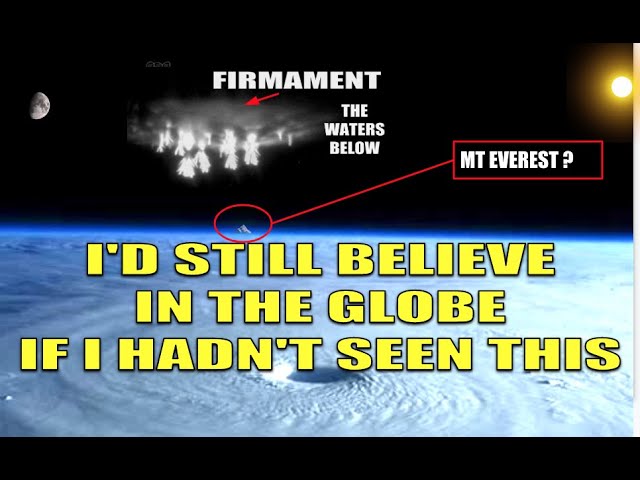The image depicts a computer-generated scene set in space with a solid black background. On the left side, part of the moon is visible, while the right side features a bright yellow circle representing the sun. Dominating the top center portion is the word "Firmament" in white letters, accompanied by a red arrow pointing downward to a cluster of small white figures that appear to be wispy and cloud-like. Just below "Firmament," it states "the waters below."

The bottom half of the image showcases the surface of a blue and white planet, possibly Earth. Across this planetary surface, in large yellow letters, the caption reads, "I'd still believe in the globe if I hadn't seen this." In the upper right portion of the planet, a red-outlined box contains the text "Mount Everest?" with a line pointing toward a marked area on the planet’s surface. The entire composition contrasts strongly against the black sky, highlighting the celestial bodies and textual elements effectively.